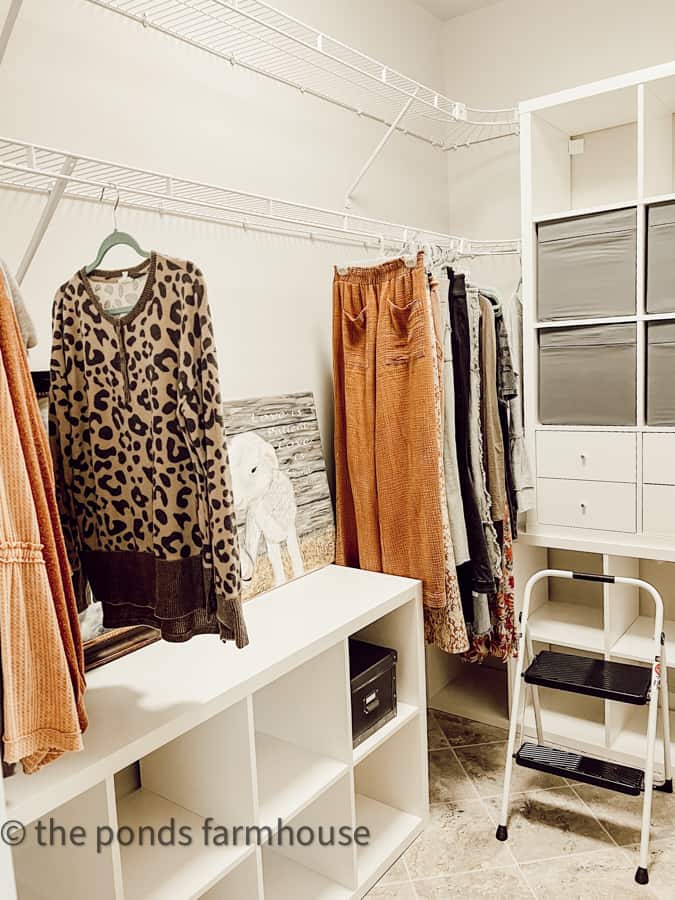The image depicts a well-organized, predominantly white closet room filled with various storage solutions and clothing items. The back wall features a built-in cabinet system with drawers, shelves, and slots designed to hold baskets or other items, with a prominent cabinet against the wall. There are two layers of wire racks; the upper rack extends farther than the lower one. Clothing on the racks includes a dominant brown and tan leopard print shirt and an orange-hued pair of pants. The tan-colored tile floor supports a two-step black and white footstool, which stands out as an immediate detail. In the lower left corner of the image, a sign reads "The Pond's Farmhouse." The room also contains a table with cubicles, one of which houses a metal box. The overall impression is of a meticulously maintained closet featuring a mix of practical storage and diverse clothing items in various colors.